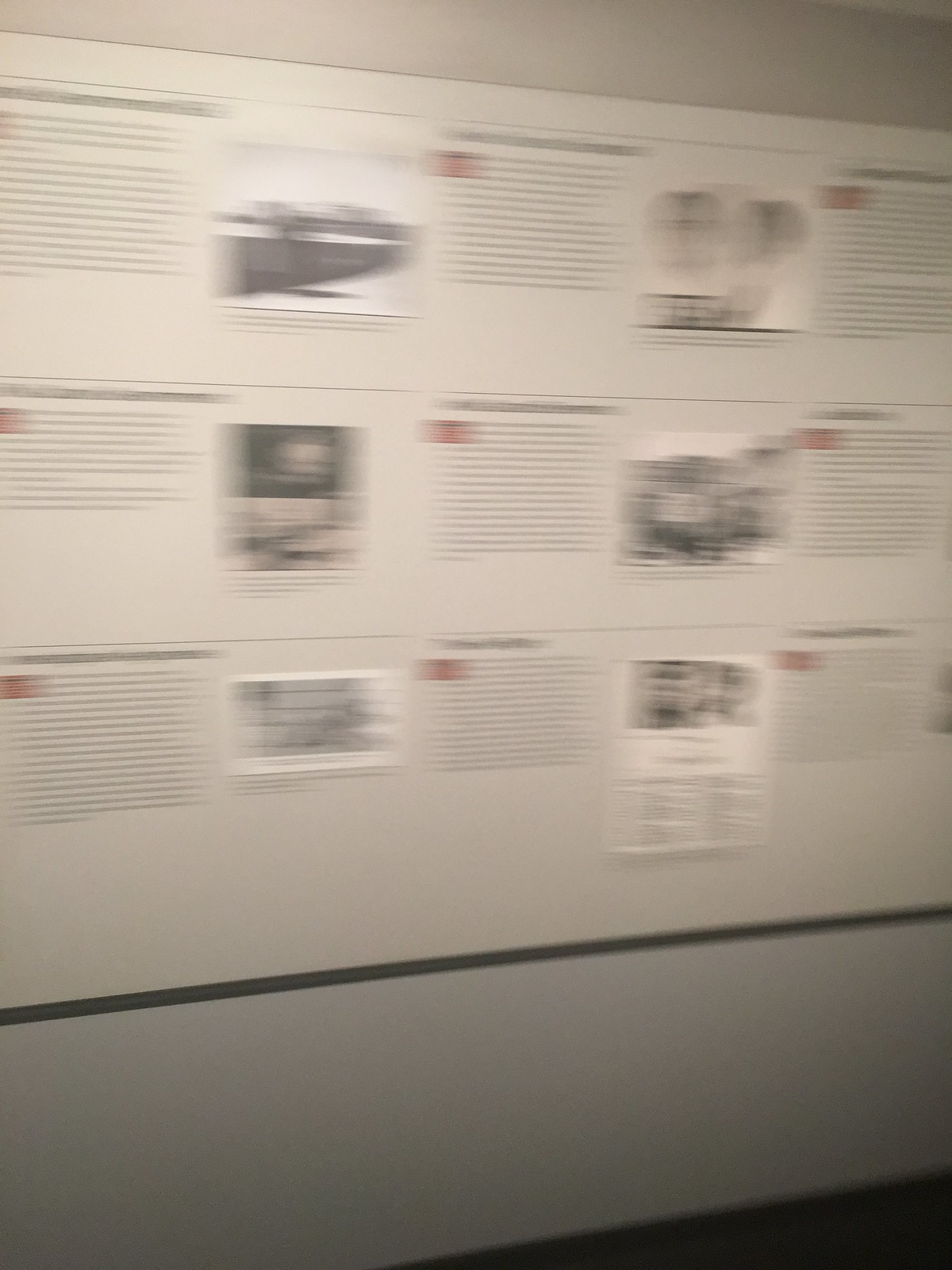In this image, despite its blurriness, one can discern a predominantly white wall adorned with a variety of elements. There are several framed pictures, each accompanied by text that extends detailed descriptions or annotations next to them. Among the images, a boat and possibly a fan can be identified, along with other assorted subjects. The wall is densely populated with text, including multiple paragraphs that provide additional context or information. At the bottom of the display, a distinct black line runs horizontally across the wall, creating a boundary or separation from other elements.